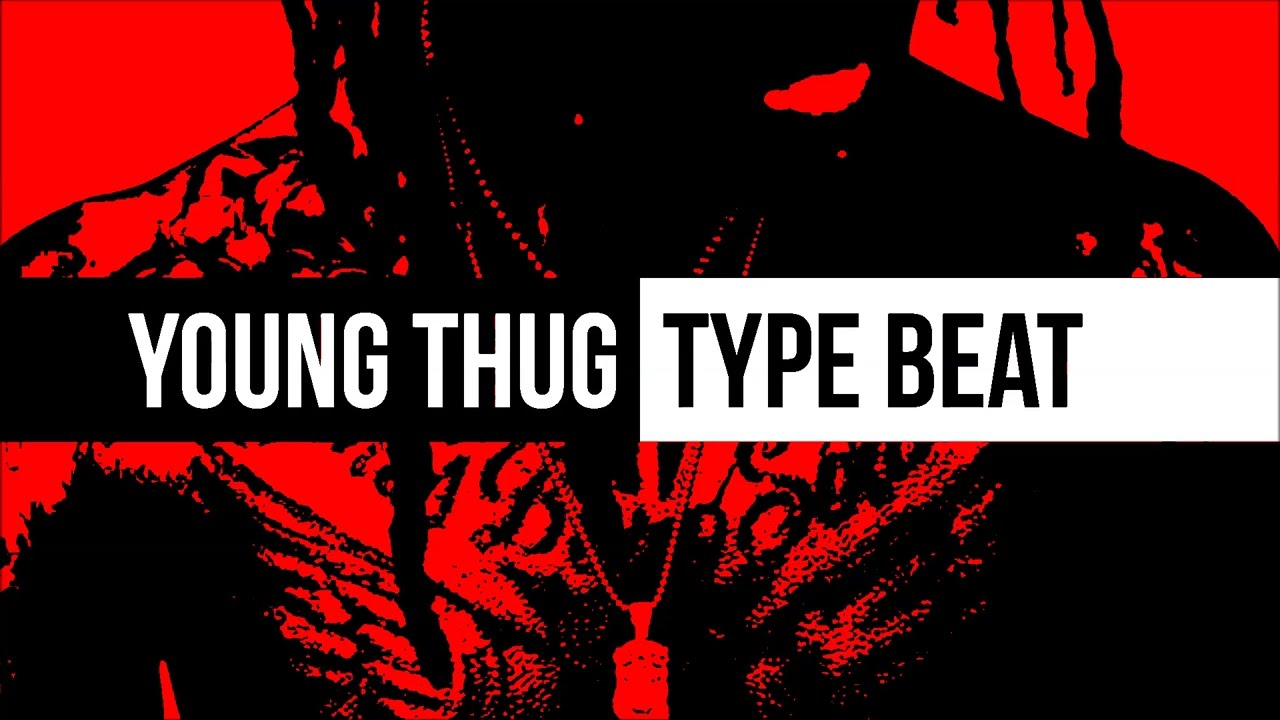The image features a minimalist graphical design with a pure black background and a centrally positioned logo. The logo's design is characterized by a prominent red ring, which appears three-dimensional due to subtle lighting and reflections. Within the ring are the capital letters "L" and "P," both rendered in an elegant, serif font reminiscent of Times New Roman. The "L" originates slightly to the left of the top edge of the ring, extending both downward and horizontally across the ring, while the "P" starts near the bottom right of the ring, extending upward and overlapping part of the ring. The letters appear to sit on top of the ring, reinforcing the three-dimensional effect. There is no additional text or imagery, focusing attention solely on the sophisticated logo design.